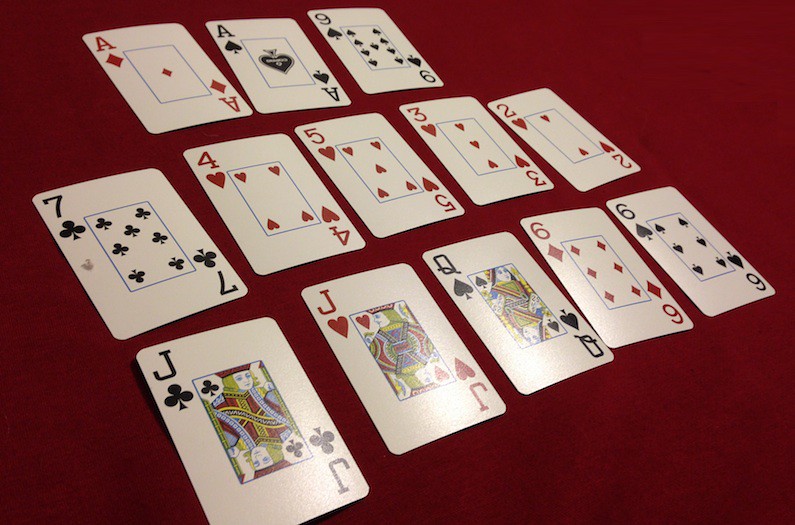A meticulously arranged collection of playing cards is displayed on a textured, red, velvet-like background, although the graininess makes it difficult to determine the exact material. The cards feature a unique design: a white background with blocky text flanking either side, while the traditional symbols of the playing cards are compressed into a small, vertical rectangle in the center. Each card's suit and rank are prominently displayed beneath its identifier, with the outlines of the central rectangles tinged in blue and the interiors remaining white.

The cards are organized into three rows. The top row consists of three cards: the Ace of Diamonds, Ace of Spades, and Nine of Spades. The second row houses five cards: the Seven of Clubs, Four of Hearts, Five of Hearts, Three of Hearts, and Two of Hearts. The bottom row also contains five cards, slightly overlapping with the second row: the Jack of Clubs, Jack of Hearts, Queen of Spades, Six of Diamonds, and Six of Spades.

Notably, the Seven of Clubs on the far left of the second row features a small gray splotch on the left-hand side. A few of the cards exhibit slight upward bends, causing them to cast small shadows to the left, particularly noticeable on the bottom left card and the Seven of Clubs above it.